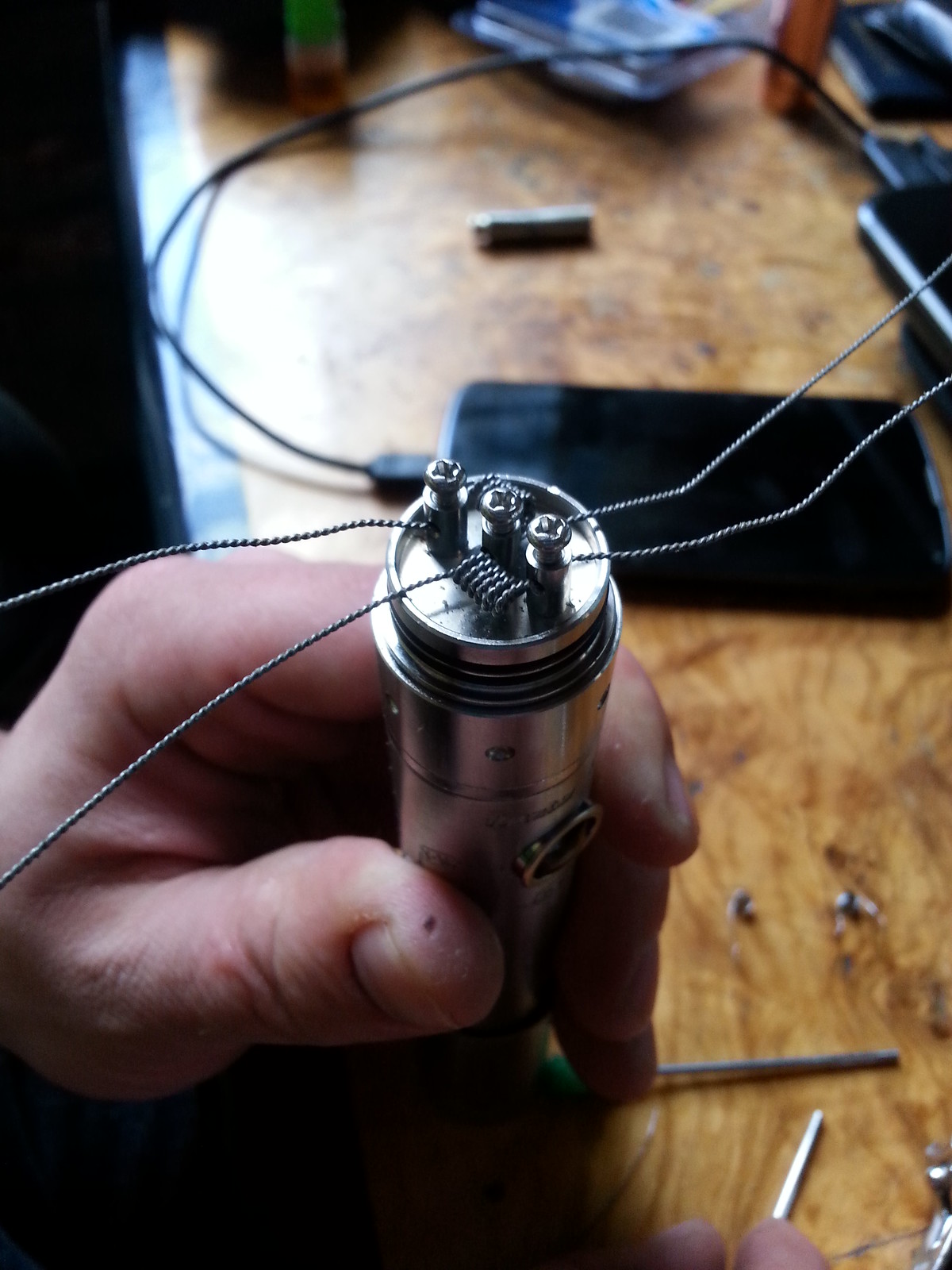The photograph captures an overhead view of a wooden workbench bathed in natural light. The central focus is on the bottom left corner, where a left hand is prominently holding a round, silver metallic cylinder. This cylinder features three vertical Phillips head screws on top, with braided metal wires extending from each screw—two wires to the left and two to the right. The fingers of the hand are wrapped around the top of the cylinder, with the thumb positioned in front, providing a secure grip.

In the mid-center of the table, there is a black smartphone placed on its side, connected to a black USB charging cable. The phone appears to be off. Scattered across the wooden surface of the workbench are several tools, loose nails, screws, and a couple of silver rods or pins adding to the cluttered, active workspace. The background elements, including some additional out-of-focus objects, contribute to the busy, functional atmosphere of a well-used workbench.